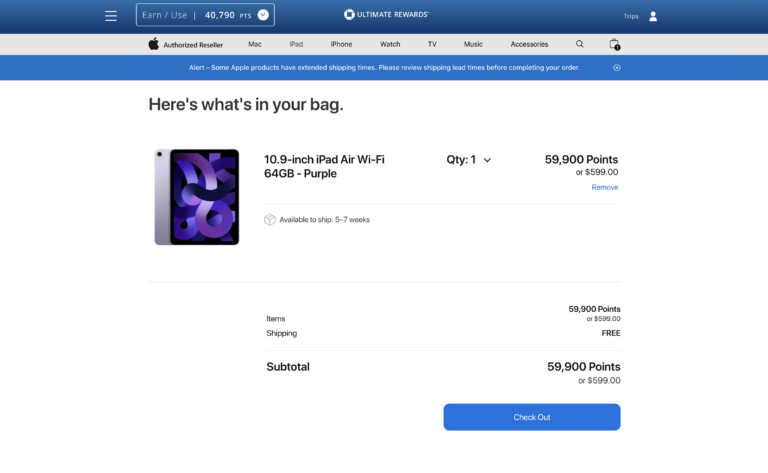At the top of the image, a long dark blue bar prominently displays "40,790 PTS" for points. To the right of this is the text "Ultimate Rewards." Moving down to the next row, there is a black apple symbol indicating an authorized reseller. Horizontally aligned next to this are the categories: Mac, iPad, iPhone, Watch, TV, Music, and Accessories. Below these categories is a long blue line.

In black text, it states, "Here's what's in your bag." Below this line, an image of an iPad screen with a black background and bold purple lines that appear three-dimensional is shown. To the right of the image, the description reads, "10.9-inch iPad Air, Wi-Fi, 64 gigabyte, Purple." Further to the right, the quantity is listed as "1" for 59,900 points. Beneath this in smaller text, it states, "or 599.00."

Towards the bottom left of the image, the word "Subtotal" is displayed, with approximately three inches to the right showing "59,900 points," and again in light gray, "or 599.00." At the very bottom, there is a blue rectangle containing the words "Check Out."